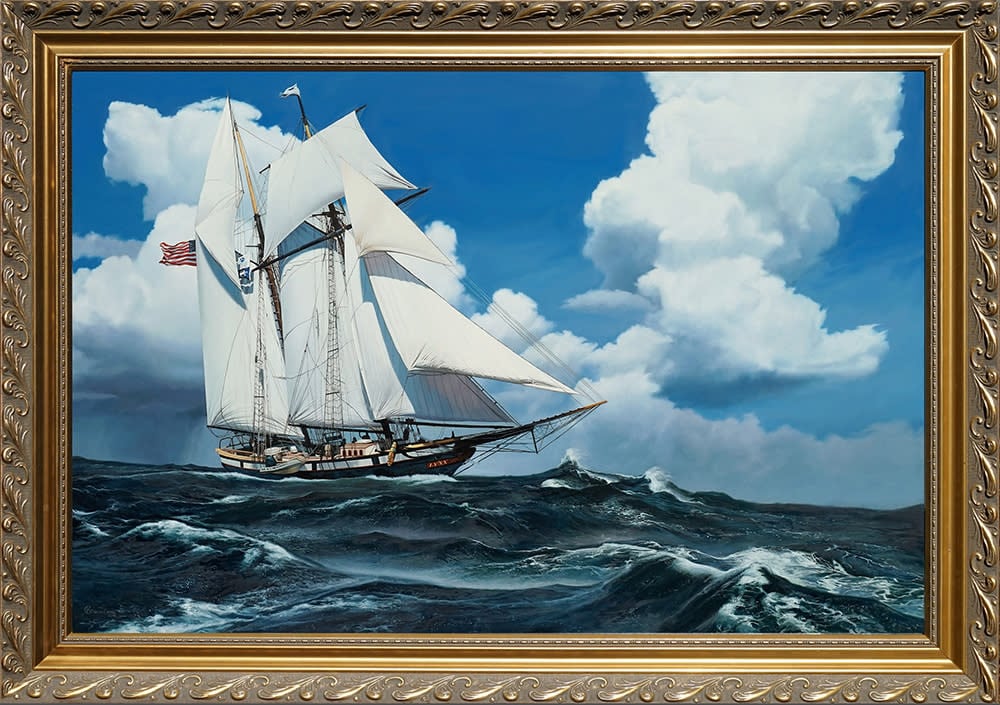This impeccably detailed, framed painting, set within an ornate, multi-layered gold frame adorned with intricate flowery designs, depicts a highly realistic ocean scene that closely resembles a photograph. Central to the image is a large sailboat, sailing on choppy, wave-filled waters with visible whitecaps and dark, rocky undertones. The sailboat, reminiscent of a historic schooner, features two towering masts with large, white sails, a complex network of rope rigging, and an American flag fluttering at its stern. The vessel's hull is striking with its blue color and prominent white stripe. Positioned right at the horizon, the sailboat stands against a backdrop of a bright blue sky, scattered with both grand nimbus clouds and smaller white clouds, enhancing the scene's dramatic and picturesque quality.